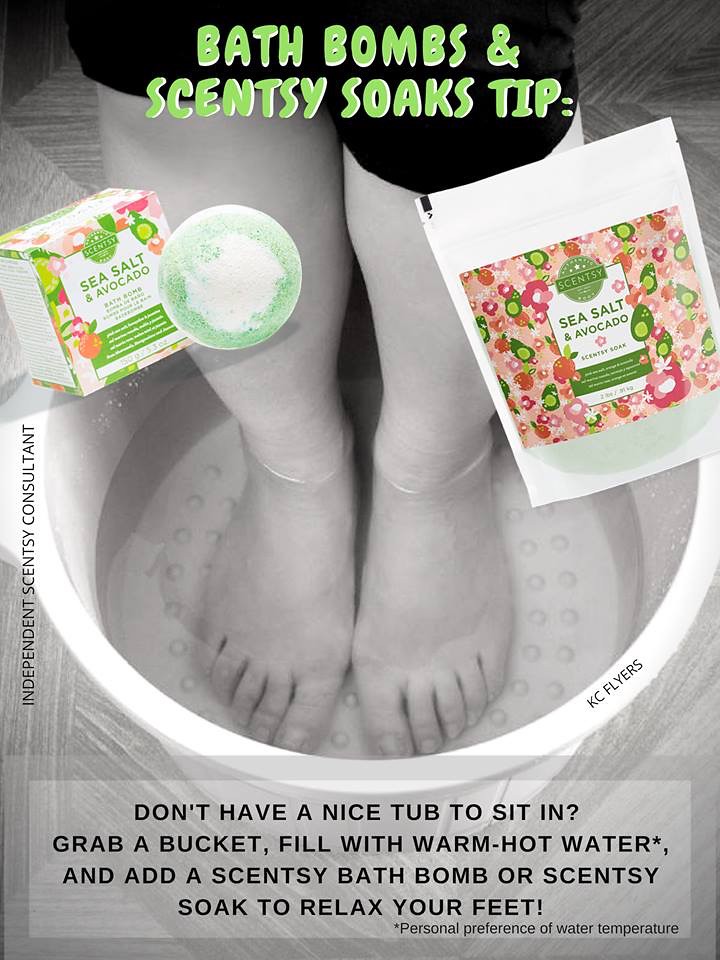The advertisement, predominantly in black and white with vibrant neon green text, is for foot bath products titled "Bath Bombs and Sinsea Soaks Tips." At the top, it reads, "Bath Bombs and Sinsea Soaps Tip," highlighting two products: sea salt and avocado bath bombs, and Sinsea soaks. These products are depicted in color, with one in a box and the other in a pouch. The ad features an image of feet being dipped in a bucket of water, emphasizing that you don't need a luxurious tub to enjoy a relaxing foot soak. The text instructs: "Don't have a nice tub to sit in? Grab a bucket, fill with warm hot water,* and add a Sinsea bath bomb or Sinsea soap to relax your feet." An asterisk notes that water temperature is a matter of personal preference, suggesting you can use cooler water if desired. Additionally, the left side of the image features the text, "Independent Sinsea Consultant," alongside the label "KC Flyers."